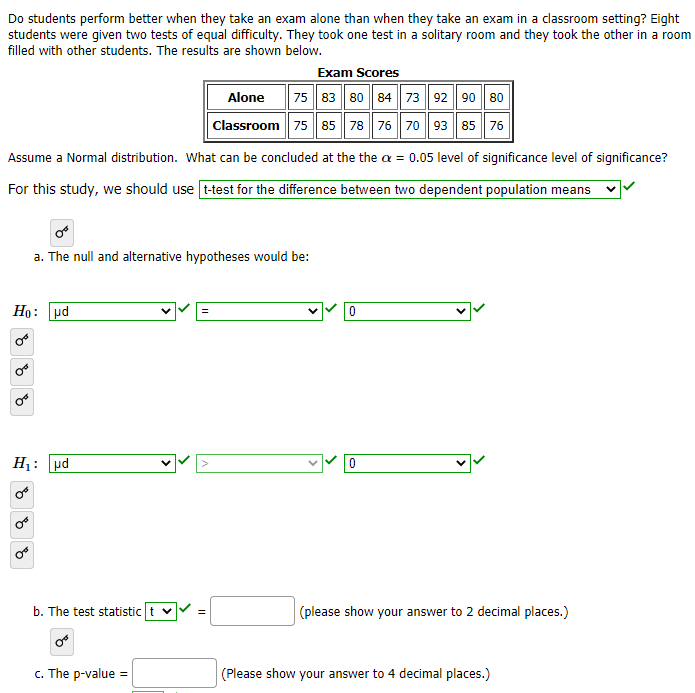The image depicts a homework assignment, likely for a math or science class, that investigates whether students perform better on exams taken alone versus in a classroom setting. At the top of the page, in black text, it reads: "Do students perform better when they take an exam alone than when they are taking an exam in a classroom setting?" Eight students were given two tests of equal difficulty, one in a solitary room and one in a classroom filled with other students. The results of these tests are presented in a chart labeled "Exam scores," with two rows of data comparing individual scores in the alone versus classroom settings. The assignment instructs: "Assume a normal distribution. What can be concluded if the α = 0.05 level of significance?" To answer the question, there's a green drop-down box that indicates using a t-test for the difference between two independent population means, accompanied by a green checkmark. Additional sections feature charts and drop-down boxes with symbols like "UD," "=", and "0," each next to green checkmarks. The interface appears to be an online questionnaire, with gray-colored buttons on the left side, and the final section at the bottom states: "The p-value equals," followed by an empty field for the answer, requesting it to be shown to four decimal places.